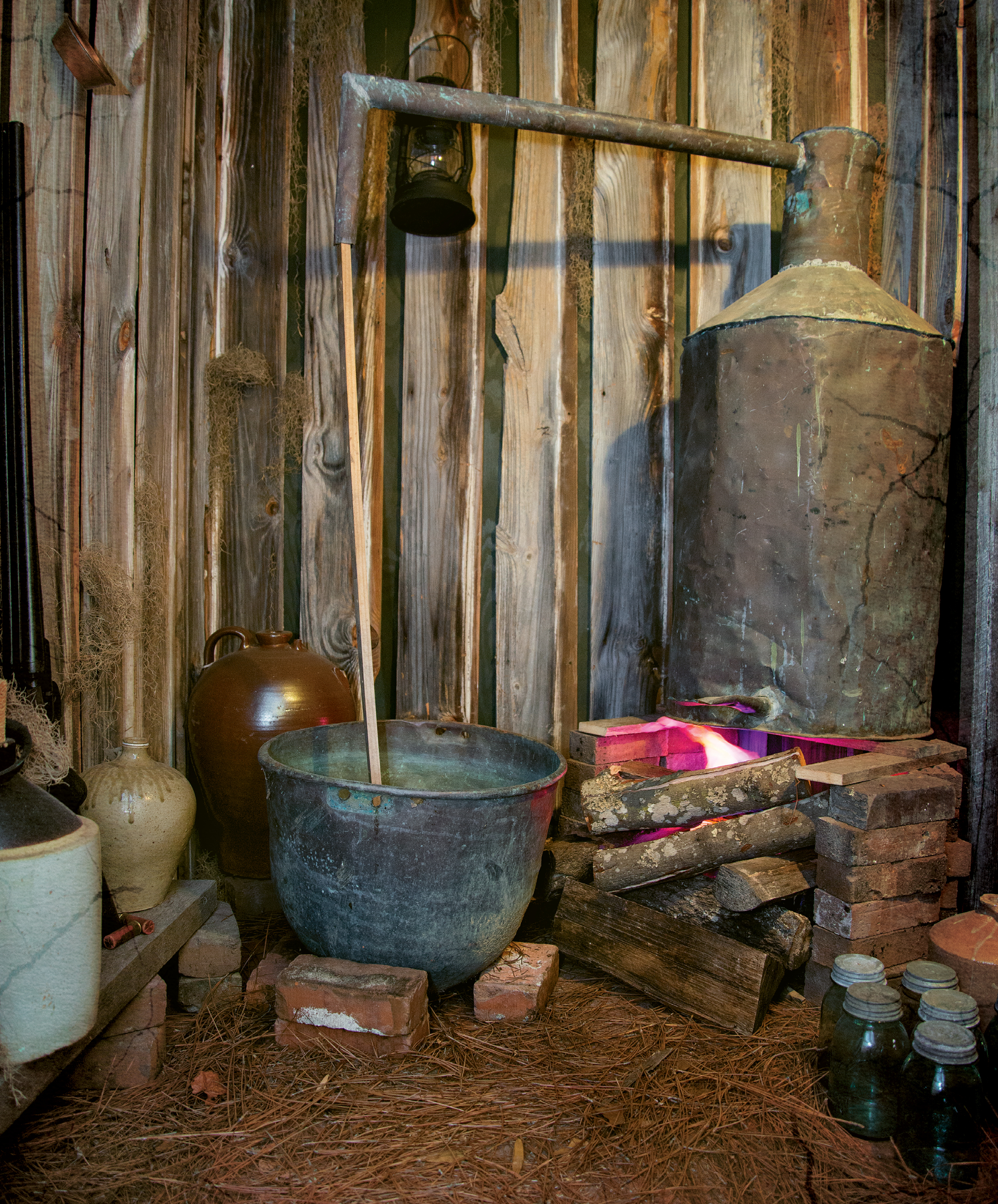The image depicts a rustic, old-fashioned setup, possibly inside a barn, indicated by the wooden walls and hay-covered flooring. Central to the composition is a large steel bucket, flanked by bricks and logs. A prominent feature is a vintage distillation apparatus. The apparatus consists of a large cylindrical chamber supported by stacked bricks, with a wooden or metal pipe extending from the chamber to a sizable copper pot positioned atop a fire. The firelight is artistically captured, illuminating the scene. In the bottom right corner, there are multiple green glass mason jars with rusted metal lids, likely once white but now aged and dirt-streaked. The ground is littered with grass and leaves, adding to the rustic, antique atmosphere of the area.